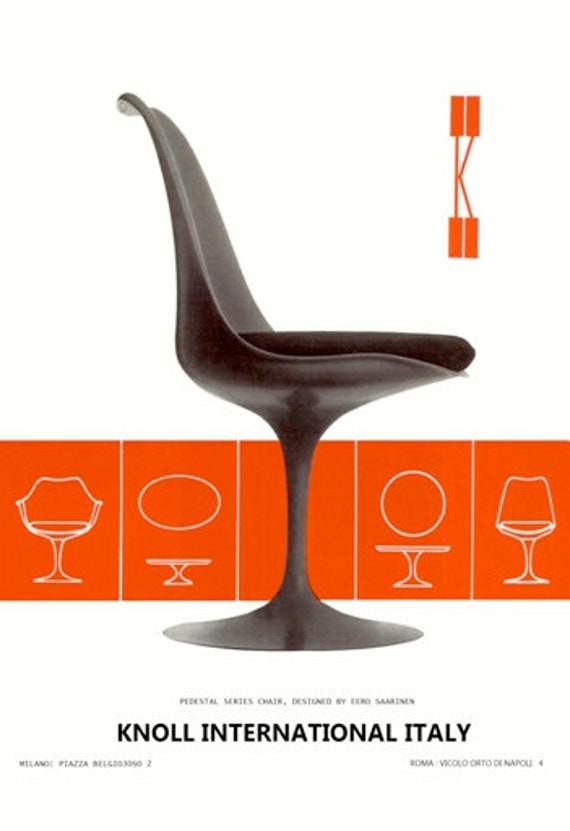The image appears to be a page from a furniture catalog or an advertisement for Knoll International Italy. Dominating the center of the page is a modern, shiny black chair that appears to be molded in one piece. This chair features a uniquely curved backrest that seamlessly transitions into the seating area, supported by a single, sleek pedestal post extending down to a round base, ensuring stability. The chair also includes a black cushion on top for added comfort. 

In the background beneath the chair, there's an orange section displaying white outlines of various chair models, including some with armrests and different base designs, depicting the different positions and variations available in this series. In the upper right-hand corner of the image, there is a distinctive red K logo with thin stems and thicker rectangles at the ends, symbolizing Knoll.

At the bottom of the image, the text "Knoll International Italy" is prominently displayed in black, with smaller, barely readable text positioned around it. Additionally, the image contains other inscriptions: "Milano Piazza" in the bottom left and "Roma Piccolo Orto de..." in the bottom right, indicating different locations, although the text is partially unclear. This well-crafted layout and design emphasize the elegance and innovation of modern furniture showcased in the Knoll International collection.